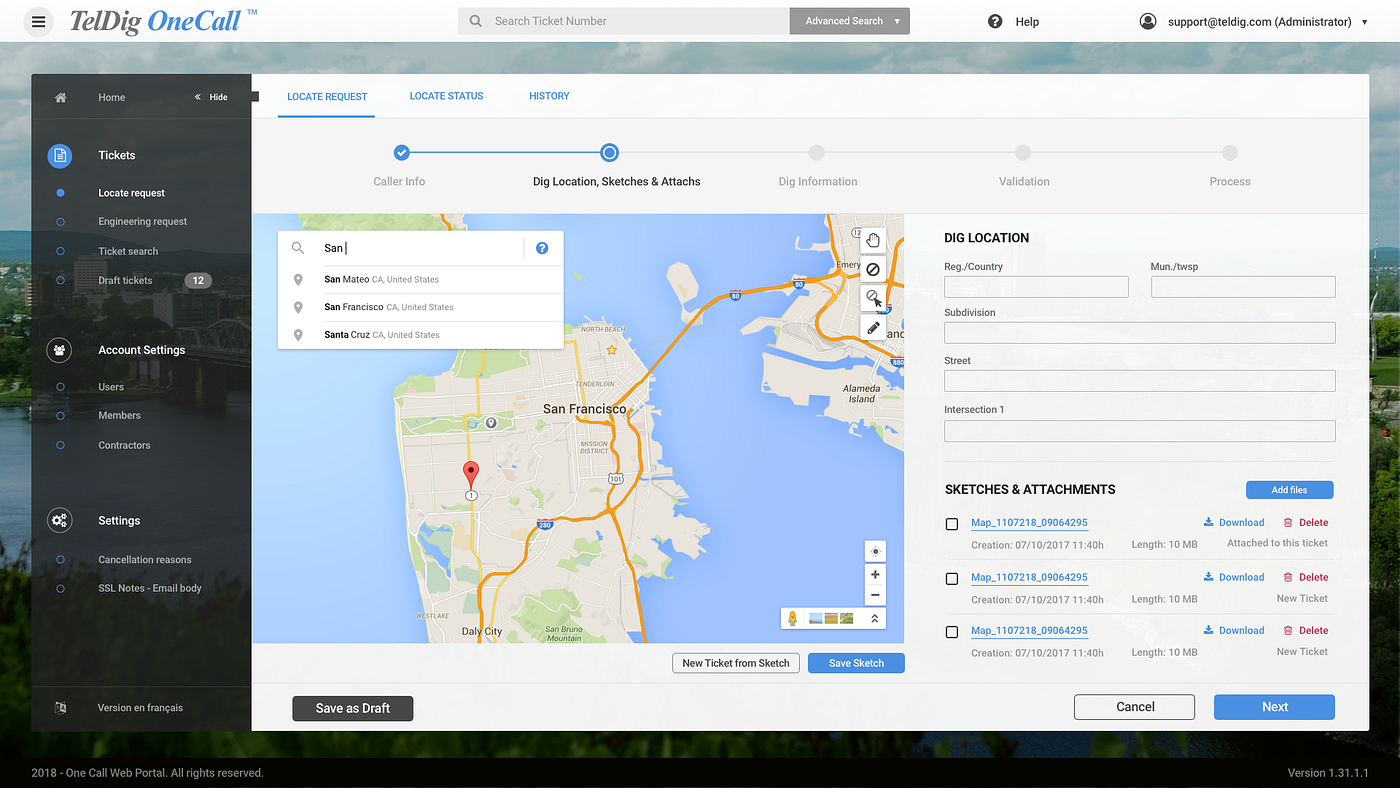Detailed Caption: 
The image depicts a web page from a service named "TelDig OneCall." The name "TelDig" is displayed in a light black or dark gray font, while "OneCall" appears in blue text, all positioned in the top-left corner. Below this header, a vertical menu bar spans the left side of the page. This menu bar includes items listed from top to bottom: "Home," followed by "Tickets" which features a blue circular logo to its left, then "Locate Request," "Engineering Request," "Ticket Search," and "Draft Tickets."

The central section of the web page displays a map that focuses on San Francisco, California. A prominent red pin marks a specific location on the map, although the exact address is not specified. The interface seems similar to that of a map or navigation application. Below the map, there are labels such as "Dig Location," "Sketches and Attach," indicating sections or functionalities related to the map content, possibly for managing excavation requests or related activities. The overall layout suggests that the page is used for coordinating excavation or engineering tasks in specific geographical areas.